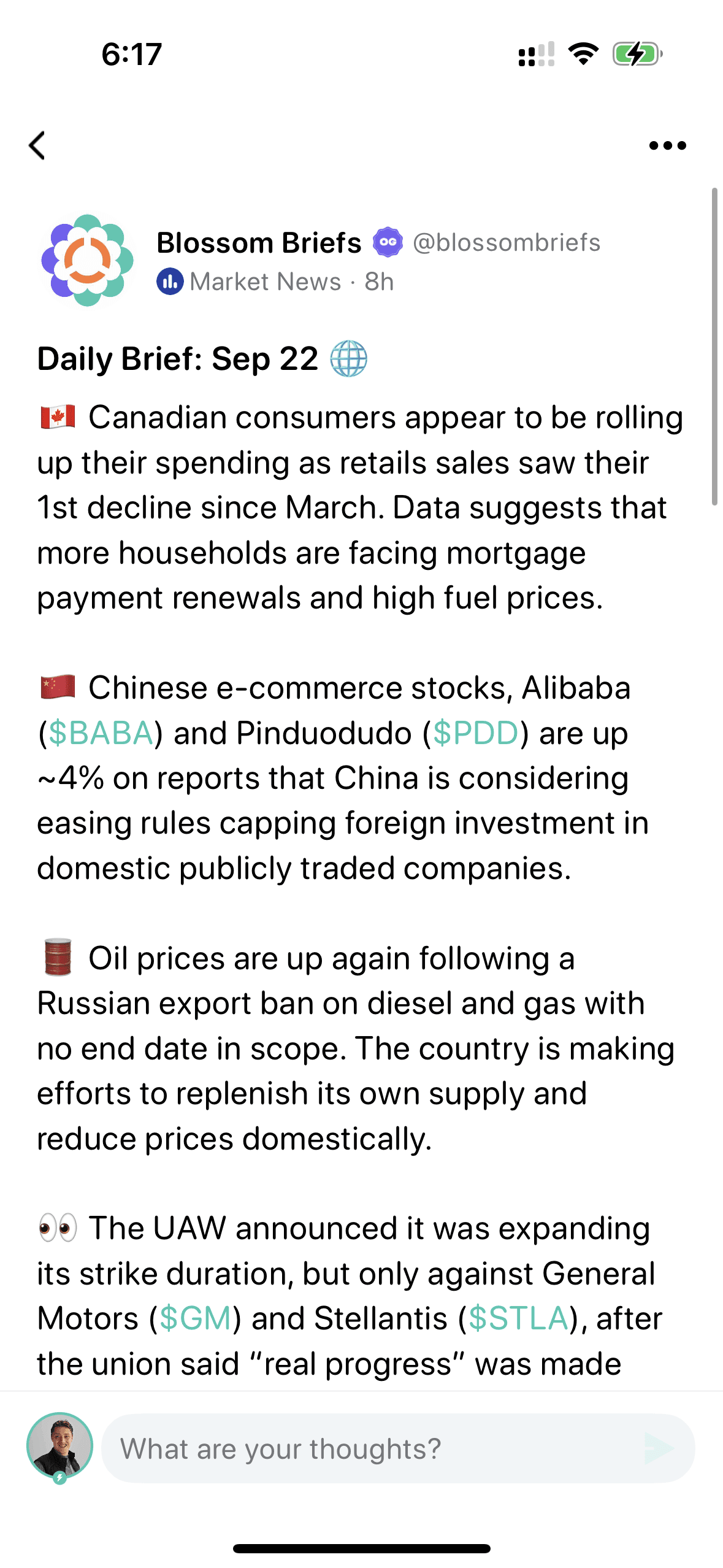Screenshot of the "Blossom Briefs" Market News Summary: 

Dated September 22nd, this daily brief provides succinct updates on key market developments from the past eight hours. The summarized stories include:

1. **Canadian Retail Sales**: A notable decrease in consumer spending as retail sales drop for the first time since March.
2. **Chinese E-Commerce Stocks**: Significant gains for major players like Alibaba and Pinduoduo, with stock prices rising approximately 4%.
3. **Oil Prices**: An increase in oil prices driven by Russia's export ban on diesel and gas.
4. **United Auto Workers Strike**: An announcement on the expansion of the strike by the United Auto Workers.

Blossom Briefs delivers these updates directly to users' phones, aiming to provide concise market-relevant information that informs about various financial movements and trends. 

At the bottom of the brief, there's a picture of a man accompanied by a text box asking, "What are your thoughts?" to encourage user interaction and feedback. Despite the absence of additional links or detailed articles, this interactive element offers a space for users to express their opinions on the briefed stories.